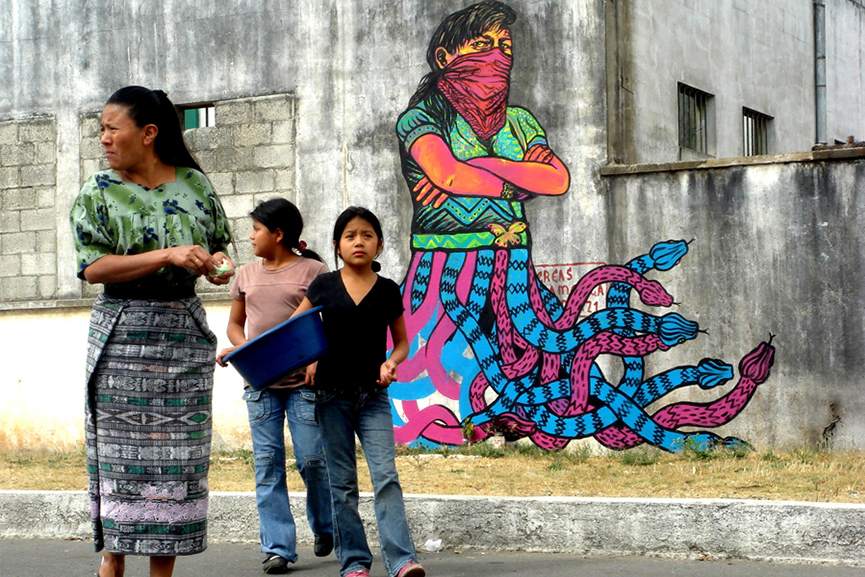In this vibrant and detailed outdoor photograph, three individuals stand on a dirt and gravel area in front of a striking mural painted on a gray concrete wall. The mural is a colorful and intricate piece, featuring a central figure with a human upper body, adorned in a green and blue striped shirt and a purple bandana covering most of the face, while the lower body morphs into an array of blue and pink snake-like creatures, with about ten serpents extending downward. 

On the left side of the image, a woman in a dress paired with a white and green shirt gazes to the left. Accompanying her are two young girls, both dressed in jeans and short-sleeved shirts. One of the girls, positioned at the front, holds a blue plastic bucket in her hand. The group stands near a grassy patch at the base of the mural, which serves as a vivid contrast to the artistic creation behind them, full of dynamic colors such as green, pink, and blue. The setting, though dominated by the mural’s intricate design, is grounded in the everyday simplicity of dirt, grass, and concrete.